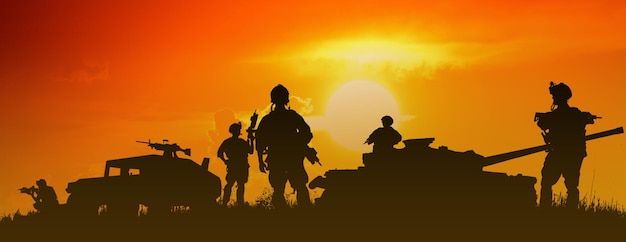In this dramatic sunset scene, silhouetted against a vibrant sky of oranges, yellows, and reds, a formidable military ensemble commands the landscape. Dominating the right side of the image is a tank with its gun extended, atop which sits a soldier brandishing a firearm. Beside the tank, another soldier stands clad in body armor. Between this robust machine and a Humvee, which is stationed to the left with a machine gun mounted atop, are two more silhouette soldiers; one raises his gun in the air, while the other holds his to the side. On the far left, next to the Humvee, a crouched soldier peers through the scope of his gun, ready and vigilant. This striking photograph captures the essence of military readiness, framed beautifully by the ethereal glow of the setting sun directly above the tank. The ground is adorned with the delicate outline of grass, enhancing the scene’s stark, yet poignant, realism.